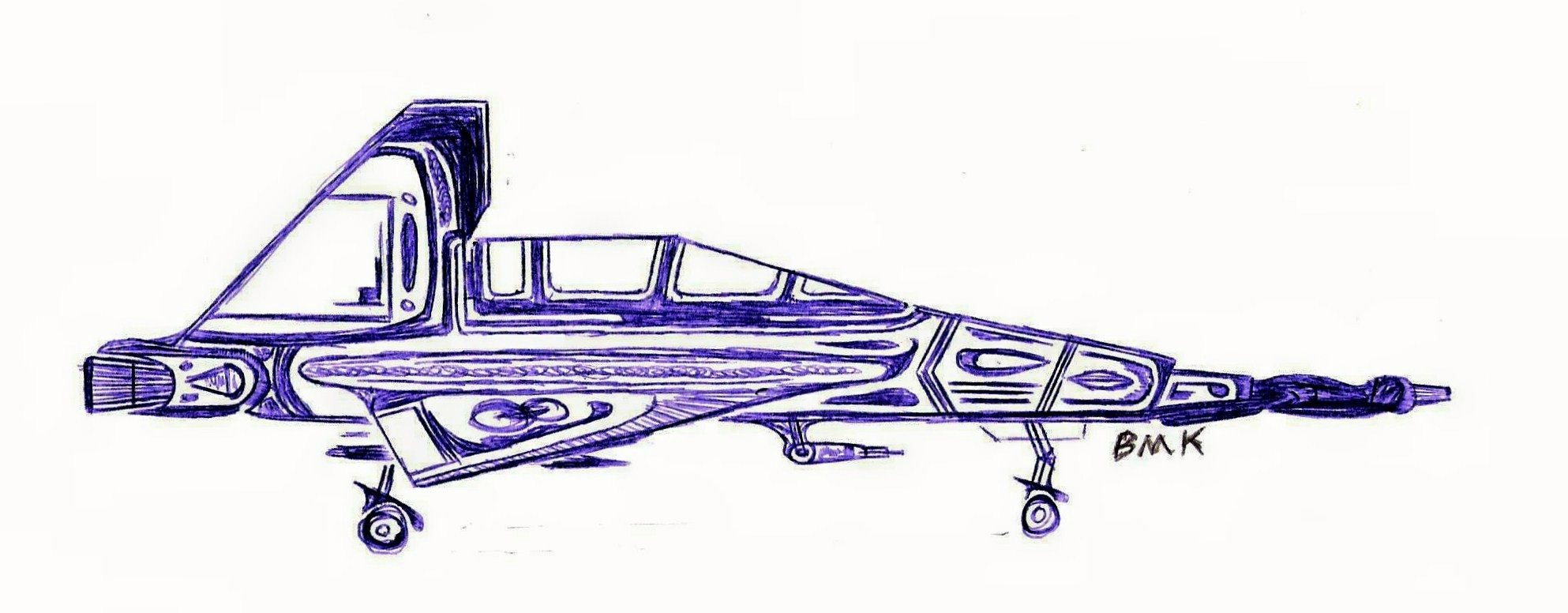This detailed pen drawing depicts a futuristic, triangular-shaped spaceship shown in a side view, facing to the right. The spaceship is primarily rendered in black and purple ink, with the black used for the outlines and the purple for details and slight faded areas. The front end of the ship comes to a sharp point, transitioning from dark purple to light purple at the nose cone. Underneath the ship, behind the front wheel but prominently visible, is a laser weapon. The initials BMK, penned in black ink, are situated to the right of the front wheel.

The spaceship features two visible triangular wings with a distinctive symbol; the wing displays what appears to be a motif resembling either a moth or two fruits connected by a black and purple spot. The body of the ship includes angular and pointy shapes throughout, enhancing its futuristic and dynamic appearance. The back of the vessel features a visible thruster and a slanted back fin that extends downward towards the tail. Overall, the ink drawing captures a unique blend of sci-fi elements and intricate details that bring this imaginative craft to life.